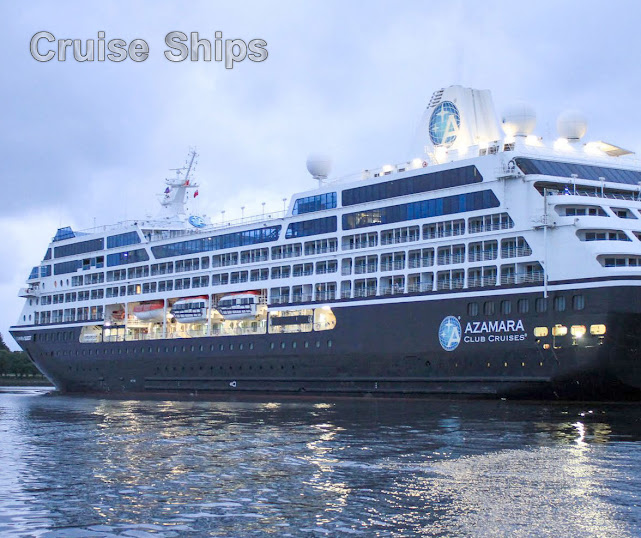A grand cruise ship named Azamara is featured centrally in the image, occupying the entire width of the frame against a backdrop of rippling water and a cloudy sky that suggests an impending storm. The ship, painted in navy blue with a white upper deck, displays numerous windows and lights that shine from the lower deck. Prominently displayed in large white capital letters on the side of the ship are the words "Azamara Club Cruises." Adjacent to this text is the cruise line's logo, a blue circle containing a white letter "A" flanked by two white stars. In the top left corner of the image, the phrase "Cruise Ships" appears in gray letters outlined in black, adding to the overall nautical theme. The scene is anchored by the ship's position at a boat dock, framed by hues of gray, blue, white, yellow, and red, immersing the viewer in a maritime atmosphere.